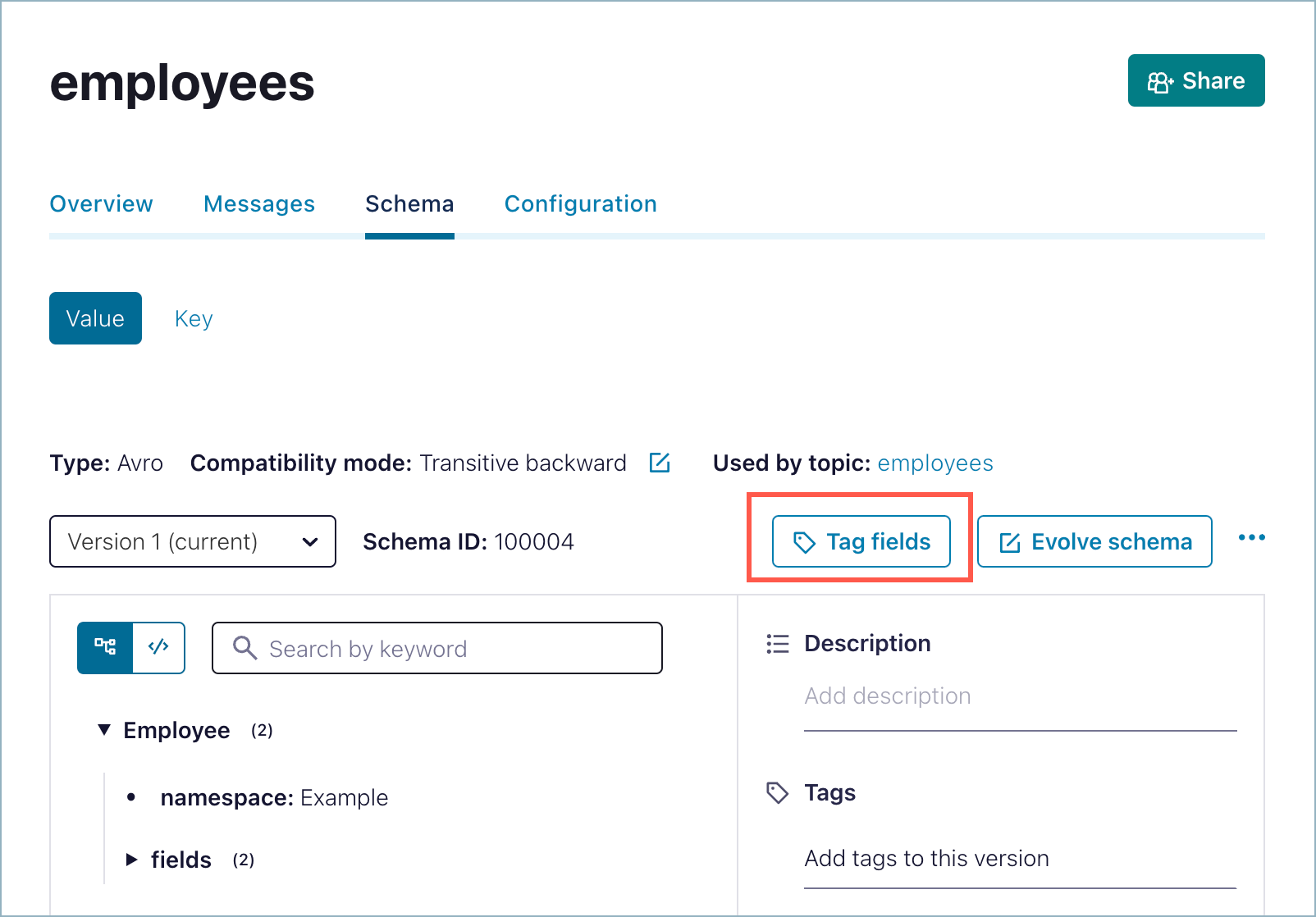This image depicts an employee-focused web page designed for internal use, where staff can log in and manage various tasks. At the top of the interface, there is a prominent "Employees" label, accompanied by a green "Share" button on the right. Just below, a set of navigation tabs includes "Overview," "Messages," "Schema," and "Configuration," with "Schema" currently highlighted.

Under the "Schema" section, two sub-options are available: "Value," which is highlighted by default, and "Key." The page provides specific details about the schema, indicating that the "Type" is Avro, with a "Compatibility Mode" set to transitive backward. Both attributes can be edited, as denoted by the edit icon next to them. It is also noted that this schema is used by the "Employees" topic.

Further details identify the current version as "Version 1," and the schema ID is listed as "100004." A "Tag Fields" section is displayed in a blue box with a tag emblem, highlighted with a red border, indicating it is the focal point. Adjacent to this is the "Evolve Schema" option, equipped with an edit button and a three-dot menu suggesting additional options.

Below these sections, a search function allows users to search by keyword within the "Employee" category. The search results include subtopics such as "Namespace Example" and "Fields," indicating the presence of two fields. To the right, there is an editable description area for users to delineate the purpose of the page. Additionally, there are fields for adding tags, likely to facilitate easier searching.